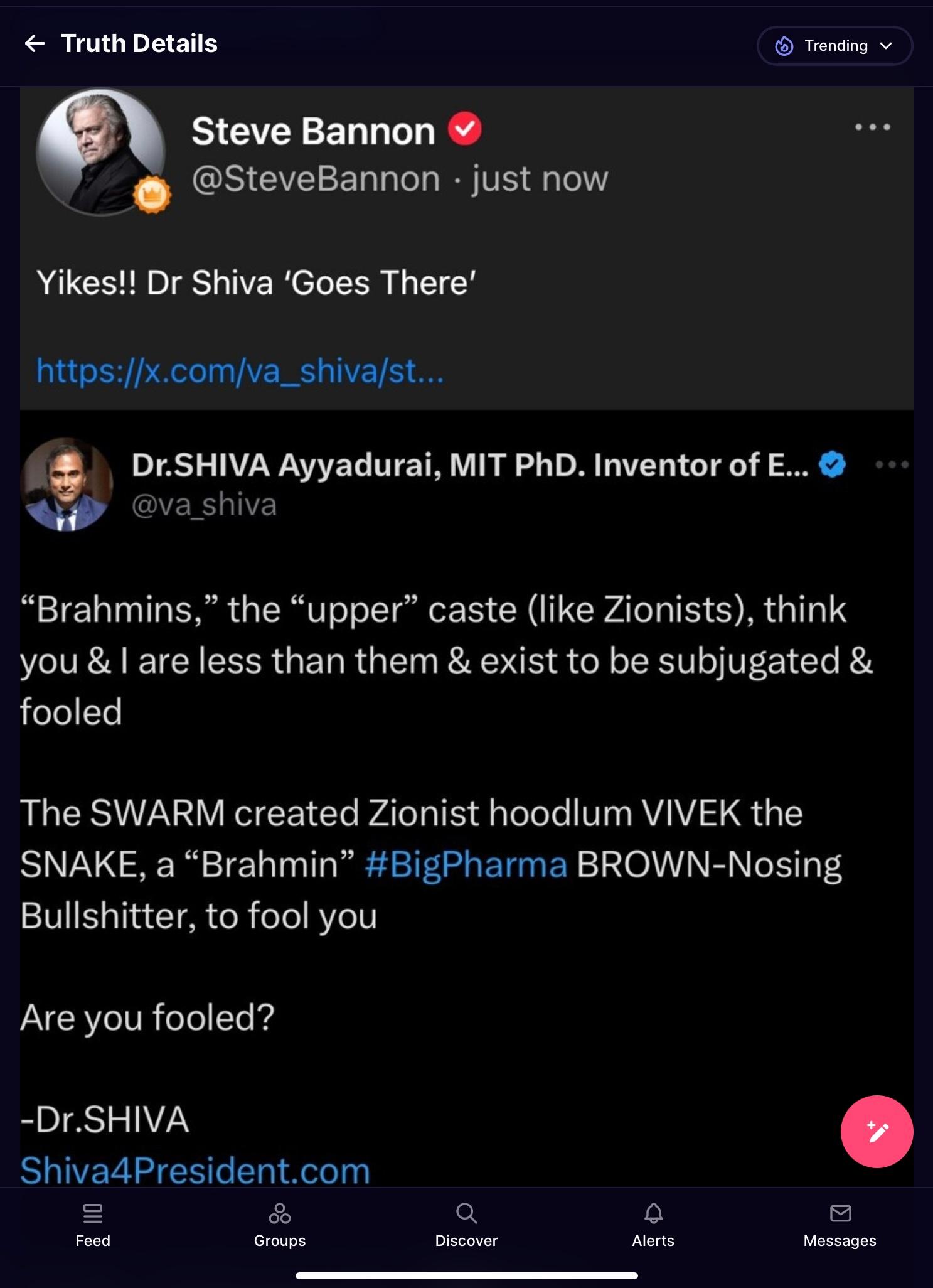This image is a screenshot from a social media platform, possibly Truth Social, displaying the account page of Steve Bannon. The account is verified, indicated by a red circle with a white tick next to the username, and the user handle is @SteveBannon. Steve Bannon's recent post reads, "Yikes, Dr. Shiva goes there," followed by a blue hyperlink.

Below Steve Bannon's post, there is a repost from Dr. Shiva Ayyadurai, who holds a PhD from MIT. His post states: "The upper caste Zionists think you and I are less than them and exist to be subjugated and fooled. The swarm created Zionist hoodlum be back the snake a Brahmin #BigPharma brown nosing bullshitter to fool you. Are you fooled? - Dr. Shiva" The post includes a link to Shiva's campaign website: ShivaForPresident.com.

At the bottom of the screen, a navigation bar houses five icons or tabs, characteristic of social media interface design.